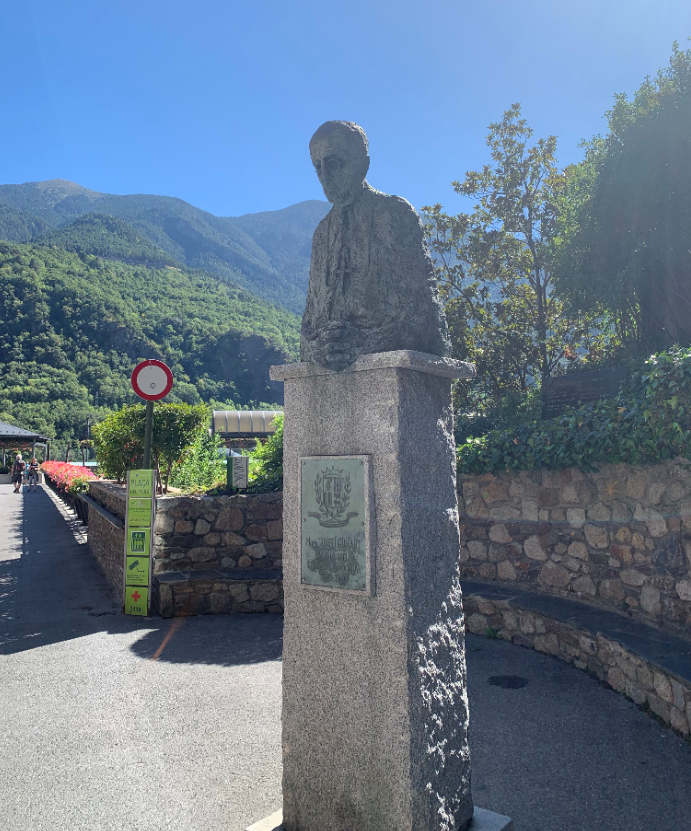The image depicts a serene memorial statue area set against a backdrop of clear blue sky and distant green mountains. The focal point is a tall gray stone pedestal with a green plaque featuring symbols, possibly including a crown and laurel leaves, although the writing is illegible. Atop the pedestal, partially emerging from it, is a somber-looking statue of a bald man, potentially light-skinned, with glasses and a large cross hanging from a chain around his neck. His hands are clasped in a prayer-like gesture. The statue, rendered in dark colors like browns and blacks, contrasts with the lighter tones of the cement podium.

The scene is enriched with vibrant greenery, including trees and bushes. To the left, a pathway leads towards what appears to be a visitor center with a blue roof. There are several people strolling along this path in the distance. The area nearer the statue includes a stone seating area with brown and black rocks, adding to the contemplative ambiance. Various small yellow signs are present, including one reading "PLAZA," accompanied by a pole featuring a white circle with a red border. The entire setting is enveloped in a gentle curvature of the road, enhancing the feeling of enclosure and reflection.